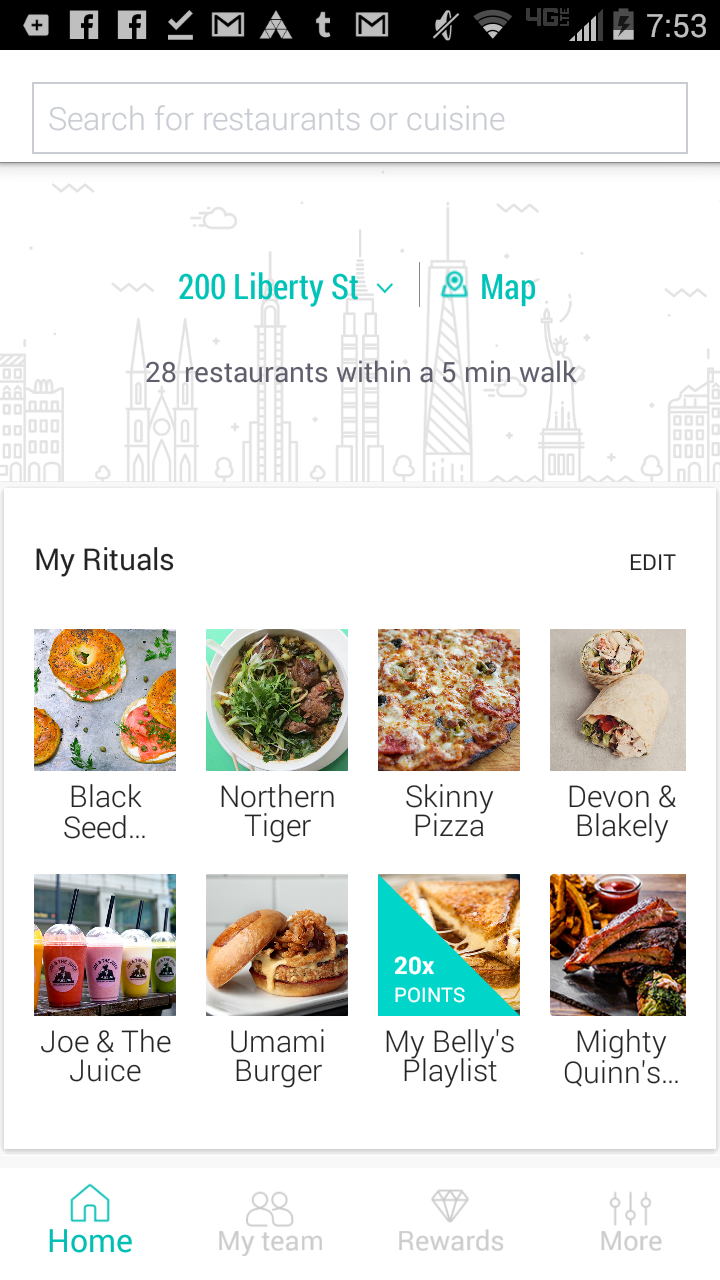The screenshot depicts a smartphone interface brimming with notifications and details. The status bar at the top reveals multiple notifications, primarily from Gmail and Facebook, along with alerts from Twitter. The phone is connected to Wi-Fi with 2 bars of signal, and it operates on a 4G network with a 4 out of 5 bar signal. The battery level is approximately one-third full, and the time displayed is 7:53.

The main section of the screen shows a search field for "restaurants or cuisine," with "200 Liberty Street" entered. There's a drop-down menu and a "map" button available. Notably, the search yields 28 restaurants within a five-minute walking distance. Below this, a section titled "My Rituals" is present, featuring an "edit" option to the right. Listed are various food options including "Black Seed Bagels," "Northern Tiger," "Skinny Pizza," "Devon and Blakely," "Joe & the Juice," "Umami Burger," "My Belly's Playlist," and "Nightly Quiz."

The bottom of the screen contains navigation buttons labeled "Home," "My Team," "Rewards," and "More." Adding a touch of personality, a doodle of a cityscape decorates the top portion of the screen behind the "200 Liberty Street" header, completing the urban theme.